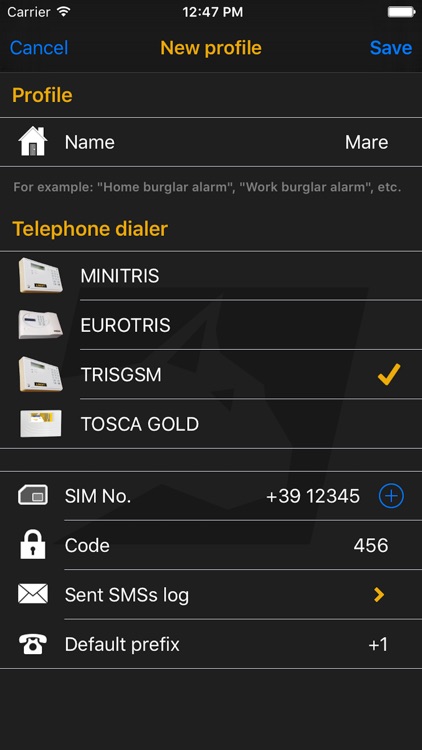The screenshot showcases an iPhone user interface, as indicated by the characteristic font and shape. In the top left corner, the status bar displays the carrier information alongside a Wi-Fi symbol. Positioned centrally, the time reads 12:47 PM, while the top right corner shows a fully charged battery icon.

Beneath the status bar, the screen features a title labeled "New Profile," accompanied by two action buttons: "Cancel" on the left and "Save" on the right. Moving further down, there's a text field labeled "Profile" where the user can input a name—currently entered as "Mare." In smaller font beneath, examples such as "home burglar alarm" and "work burglar alarm" imply this profile name pertains to a security system.

Continuing downward, the next section is titled "Telephone Dialer," presenting four selectable options. These options appear as seemingly random words like "MINITRIS," the significance of which is not immediately clear. 

The subsequent section allows for the entry of additional details including SIM number, code, an SMS log, and a default phone prefix. All these suggest customizable settings for a security system or similar application on the phone.